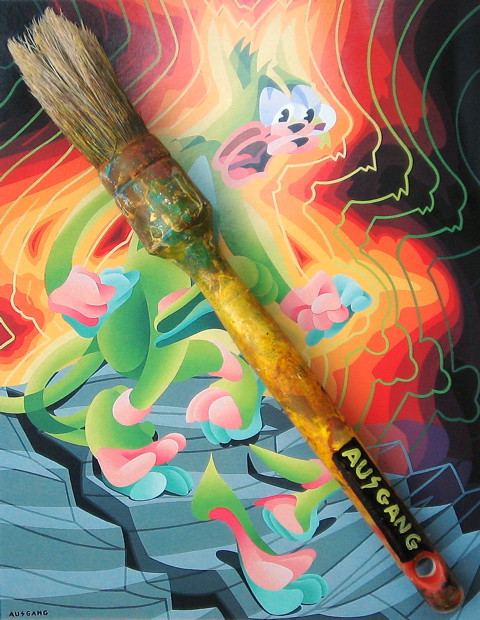This vibrant photograph features a well-worn paintbrush placed atop a vividly colorful painting. The paintbrush, with a rounded handle that transitions from yellow at the top to red at the bottom, strikes a striking pose. A black square near the bottom of the handle displays the word "AUSGANG" in bold yellow letters. The bristles, frayed from use, show remnants of old paint both at their base and where the bristles meet the handle.

Beneath the paintbrush, the artwork depicts a cartoon character poised on a staircase. The character, predominantly green with hints of blue and pink, appears to be tiptoeing down a set of gray steps. Radiating from the character are vibrant hues of orange, red, and yellow, creating a dynamic and lively scene. The character's expressive face shows open eyes and a wide mouth, suggesting movement and excitement. At the bottom left corner of the photo, the artist's signature "ASUGANG" mirrors the lettering found on the paintbrush, anchoring the connection between the tool and the art it helped create.